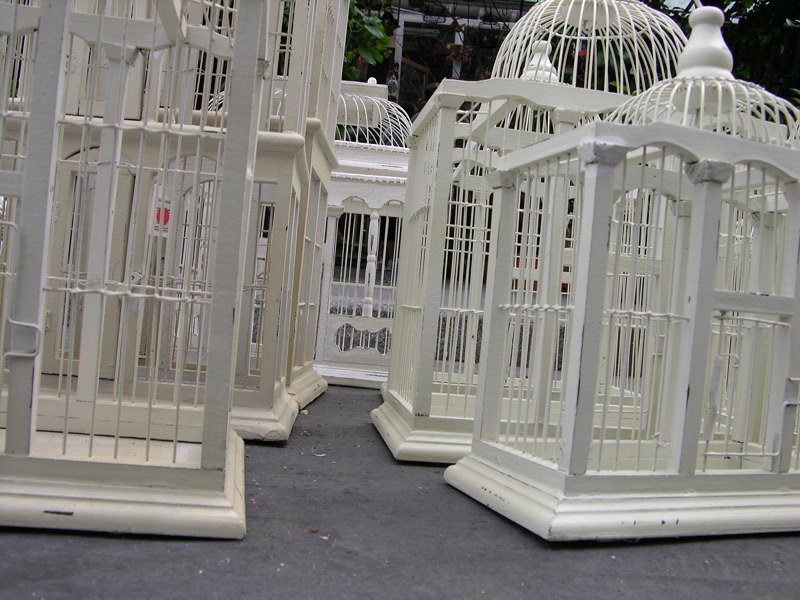This photograph captures a collection of intricately designed birdcages, arranged in an organized fashion on a gray surface, which could be either carpet or concrete. The birdcages, predominantly white in color, exhibit architectural details such as pillars and domes, resembling miniatures of grand observatories with circular tops adorned with triangular ornaments. The cages vary in size, with some being much taller than others, and they feature wooden trim at their base. Positioned on both the left and right sides, these birdcages create a small walkway down the middle of the image, leading to an additional cage at the end. In the background, subtle hints of greenery and the indistinct edge of a spacious room — possibly a studio or a pet shop — can be observed.